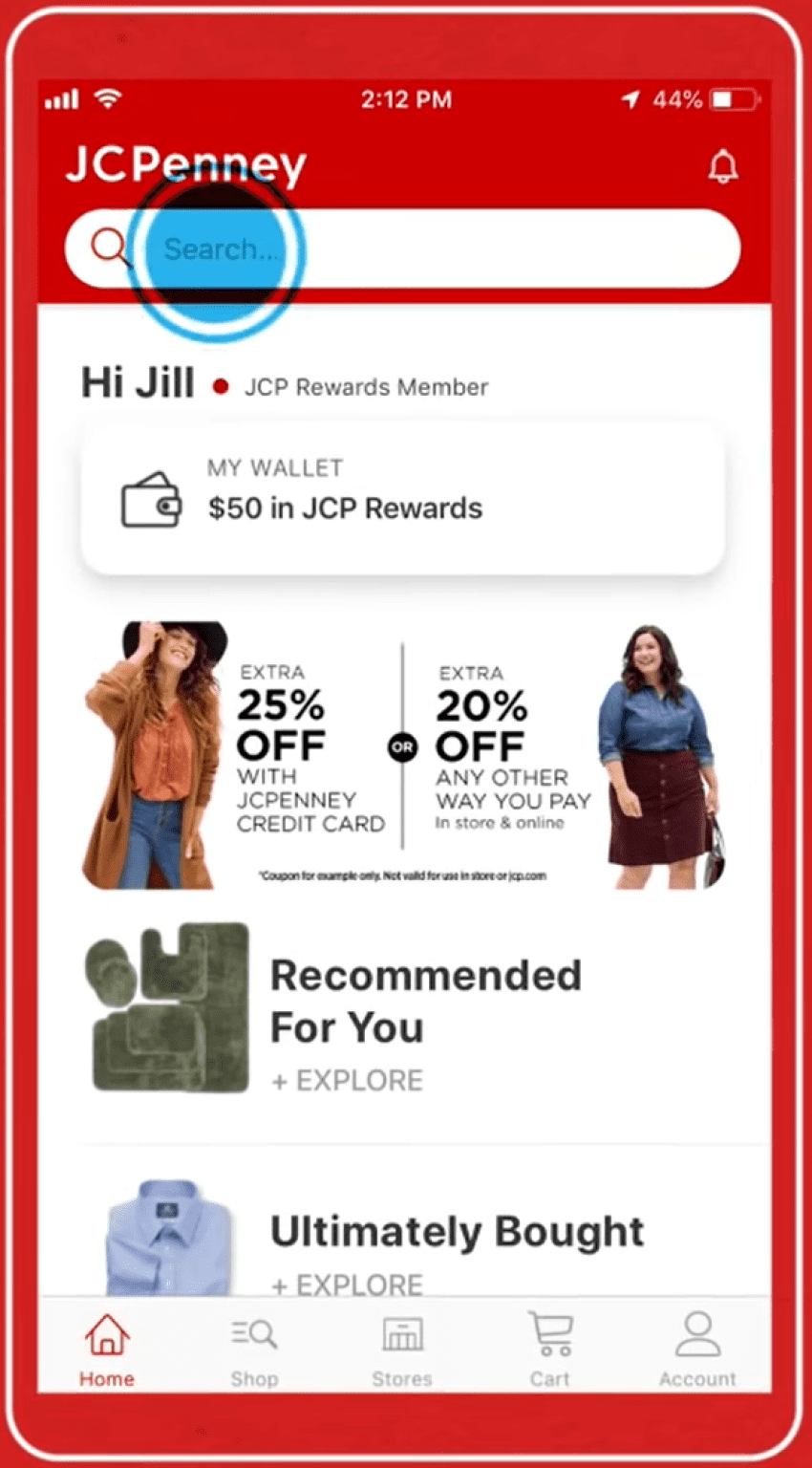Screenshot of the JC Penney mobile app.

The screenshot displays the JC Penney app interface on a red-themed phone screen. At the top, there's a prominent red bar with the "JC Penney" logo in white on the left side and a white bell icon outlined in red on the right side. Just below, the screen features a white search bar, with a red search button to the left.

Under the search bar, there's a welcome message in a white section saying "Hi, Jill" with a red dot. This indicates that Jill is a JC Penney Rewards member. Below the welcome message, there is a box labeled "My Wallet," which displays "$50 in JCP Rewards."

Further down, there's a promotional banner split into two halves by a dividing line. On the left side of the banner, a woman is wearing an orange shirt paired with blue jeans and a thick brown cardigan. The text above her states, "Extra 25% off with JC Penney credit card." On the right side, another woman is dressed in a brown skirt and blue shirt. The accompanying text reads, "Extra 20% off any other way you pay, in-store and online."

The overall design of the app is clean, user-friendly, and color-coordinated in red and white, reflecting the brand's identity.